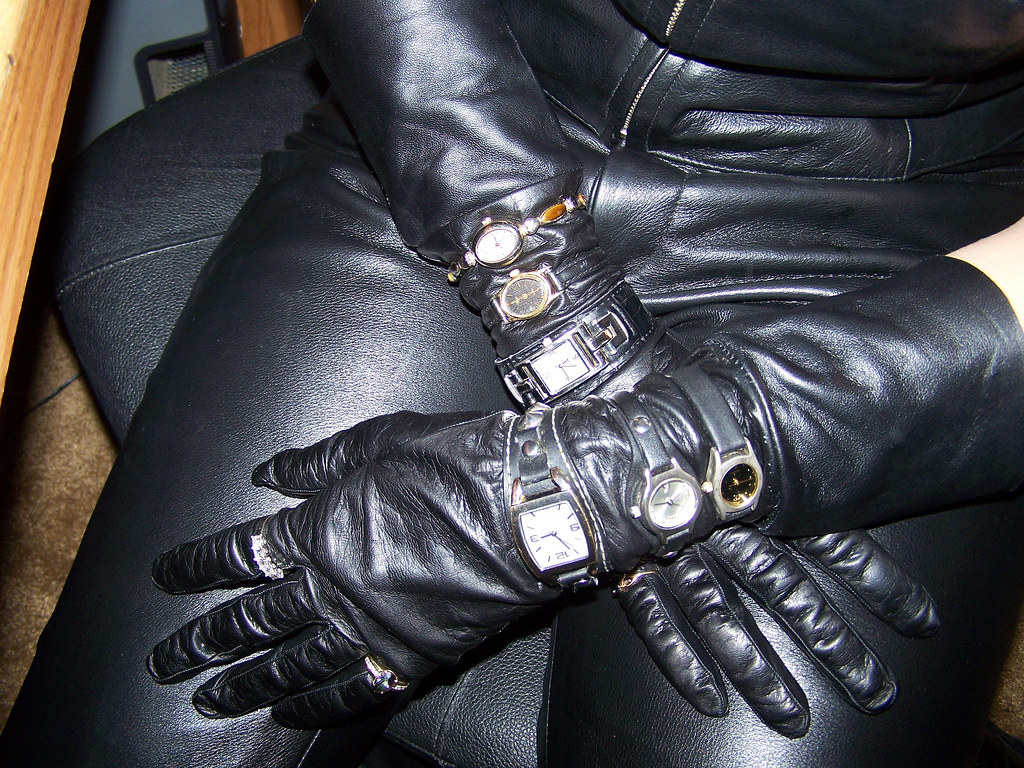In this indoor color photograph, a person sits on a black office chair, dressed entirely in black leather, including black leather gloves that extend halfway up the forearm. Looking down into their lap, with legs clothed in black leather pants, the person's right arm is draped across their thighs while the left arm crosses over it. The gloves on each arm bear three various styles of watches.

On the left arm, positioned over the glove, there are two distinctive silver rings—one on the index finger and one on the pinky finger, which also features a blue stone. The left glove displays three watches: the first, a square-faced watch with a wide leather strap closest to the hand; the second, a round-faced watch with a narrower leather band; and the third, a round-faced watch with a gold face and black leather strap.

The right glove similarly has three watches: the first, further up the arm, is a dainty watch featuring diamonds along the sides and a brown linked band; the second, a small round watch with an oblong face and a thin leather strap; and the third, a square-faced watch with a broader black band. 

Additional details include a glimpse of Caucasian skin near the elbow, the hint of a light wooden desk edge, brown carpeting, and a grayish-blue wall in the upper left corner of the image.